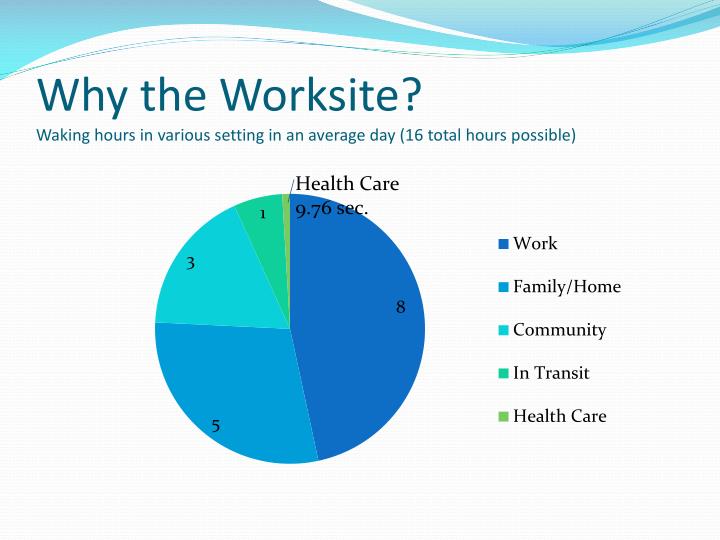The image appears to be the inside of a brochure or a poster, featuring a predominantly white background with a stylized wave design in light blue at the top. Beneath this wave, the text reads, "Why the Worksite?" followed by a subheading, "Waking hours in various settings in an average day (16 total hours possible)." Centrally positioned is a circle graph divided into various colored segments—ranging from dark blue, lighter blues to green—each representing different categories labeled as work, family/home, community, in transit, and health care. The smallest segment, labeled health care, is yellow and includes the annotation "9.76 sec." The corresponding categories and their colors are listed vertically in black text on the right side of the graph. The chart is detailed with number indicators, 1, 3, 5, and 8, within the colored segments, elucidating the distribution of waking hours across various daily activities.